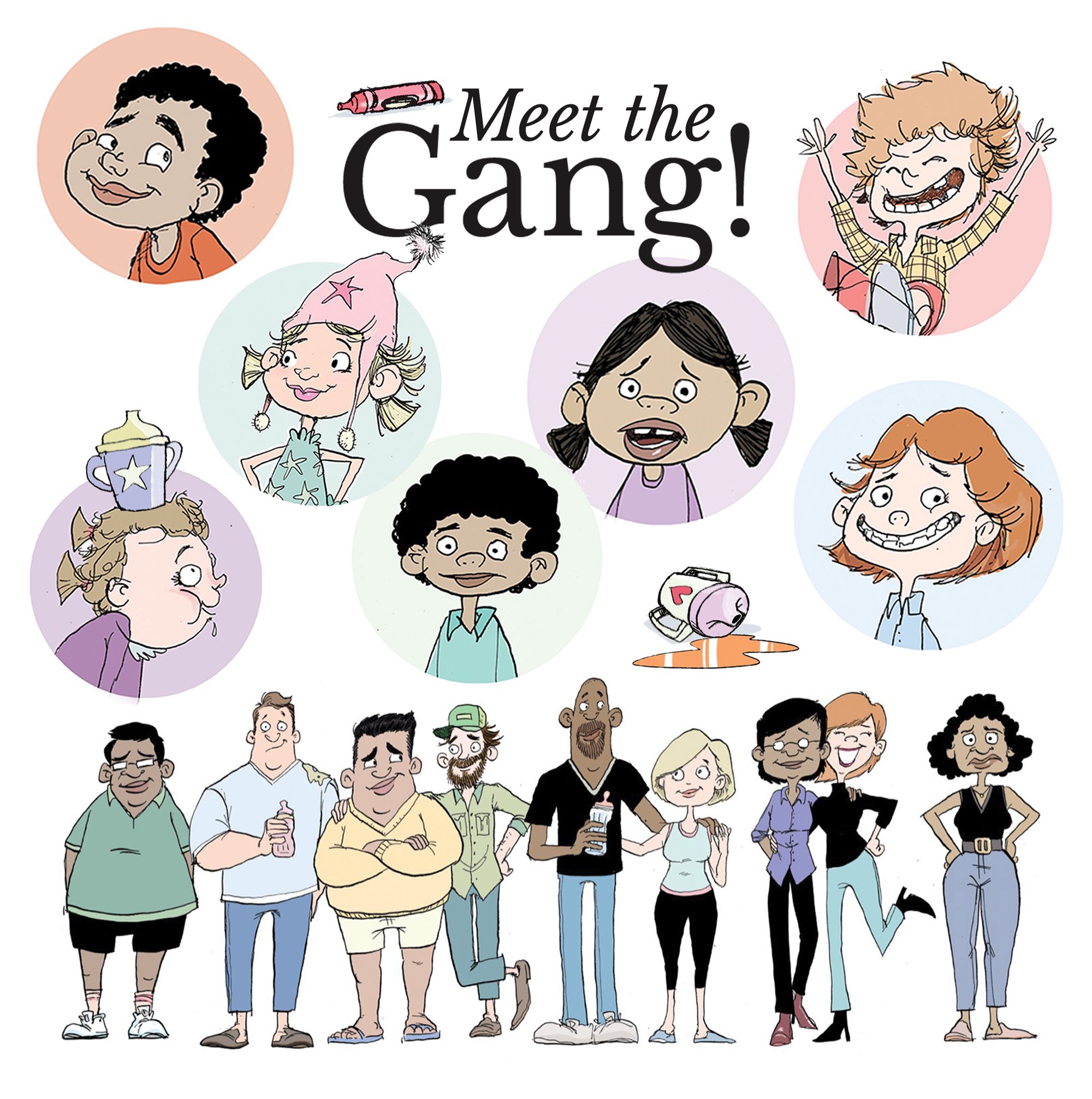This vibrant and engaging image, potentially from a children's book or cartoon show cover, features a captivating scene with numerous characters. At the top center, bold black letters announce, "Meet the gang!" with an exclamation mark, accompanied by a playful red crayon mark beside the "M" in "Meet" and over the "G" in "Gang." Below the title, seven colorful circles showcase the expressive faces of various children: a black boy in an orange shirt, an excited white girl with orange hair wearing a yellow shirt, another white girl sporting a pink hat with a star, a black girl with pigtails in a purple shirt, a smiling white girl with orange hair and braces, a black boy in a blue collared shirt, and a white baby girl whimsically balancing a sippy cup on her head. Beneath these children's portraits, their parents stand in a row, reflecting similar emotions and gestures as their kids. Some adults embrace each other, some stand with hands on hips or in pockets, and a few men hold bottles, creating a lively and cohesive family-friendly scene. A sippy cup with a pink heart and purple top spills orange juice, adding a playful touch to the setting.